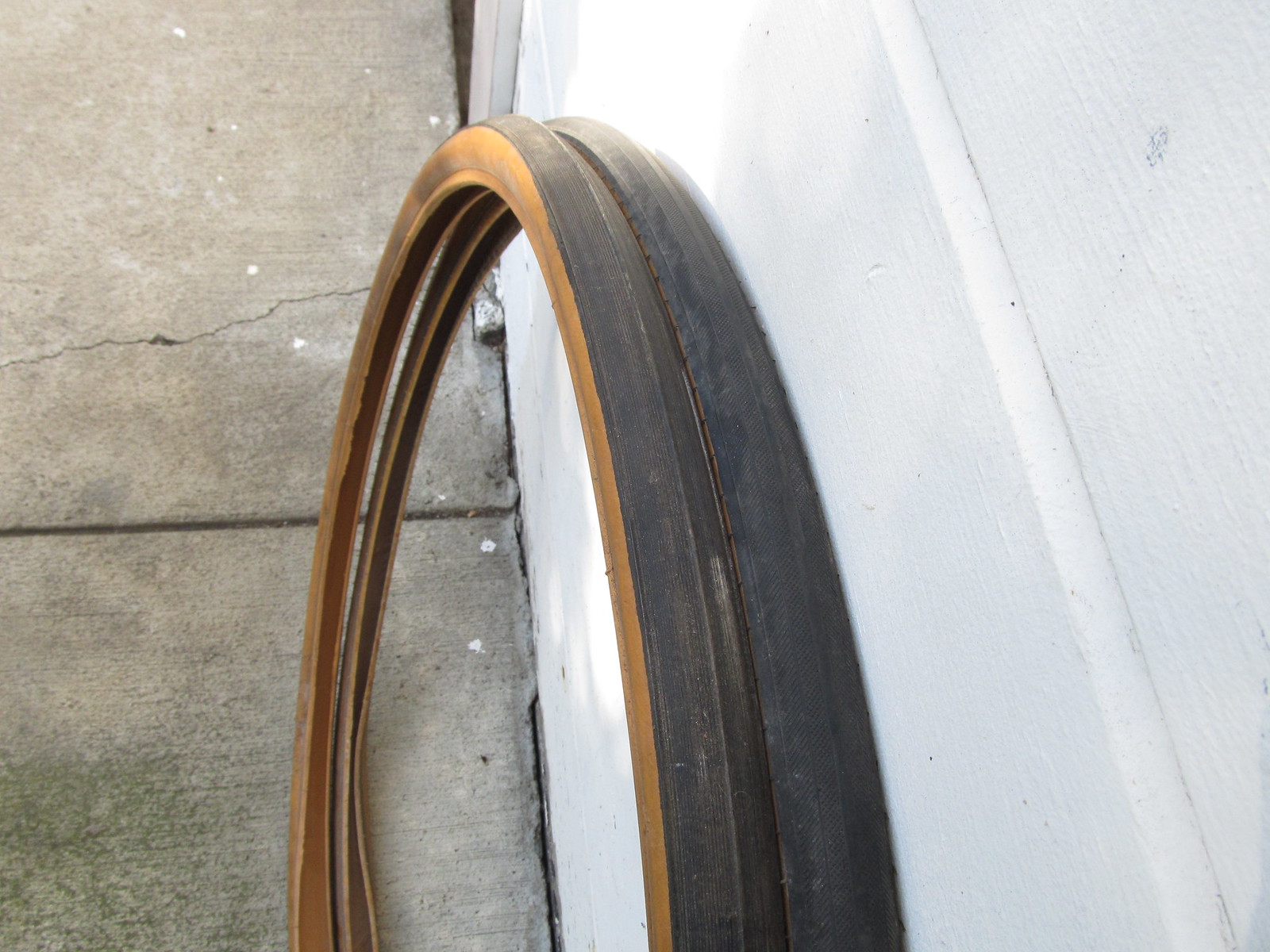The image shows two worn and hollow street bike tires leaning against a white wooden wall, likely the exterior of a house or a garage. The tires are positioned upright, with the treads extending from the bottom of the frame, curving upward before descending again, almost reaching the top of the frame. To the left of the image, there is a concrete sidewalk, which appears in shades of tan and gray. The scene is set outdoors, with the white wall and concrete providing a contrasting backdrop to the beaten-up black tires, which have no spokes.